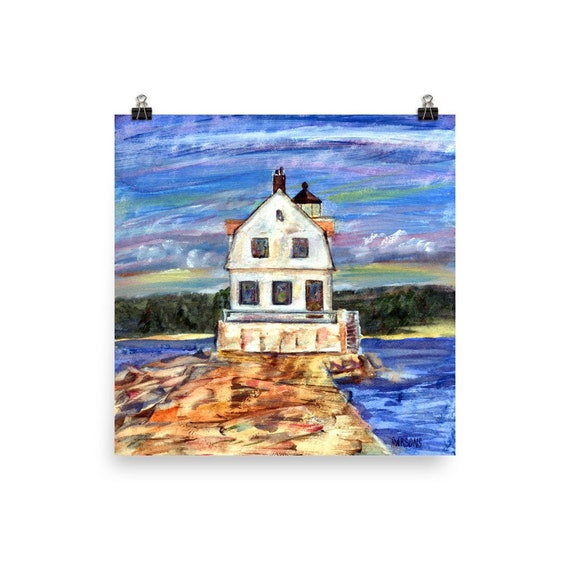The image is a beautiful watercolor painting, displayed on a white wall, suspended by two binder clips and clear thumbtacks. Dominated by shades of blues, whites, and browns, the artwork vividly portrays a large, two-story, barn-shaped house with New England-like white siding and brown-trimmed windows and doors. A chimney crowns the sloped roof, and a prominent deck or porch is visible at the front. Steps lead up to the deck, drawing attention to the inviting facade. The house, possibly a lighthouse given the peeking structure behind, is set against a backdrop of a serene body of water—perhaps a lake or an ocean inlet. The water is depicted in various shades of blue, creating an illusion of waves. In the background, a rocky, wooded terrain with evergreen trees blends seamlessly into a beach with yellow sand. Above, the sky transitions through a spectrum of colors—deep blues, light purples, and whites, with hints of green and yellow, mimicking the glow of a setting sun, interspersed with multicolored clouds, adding a captivating charm to the scene.